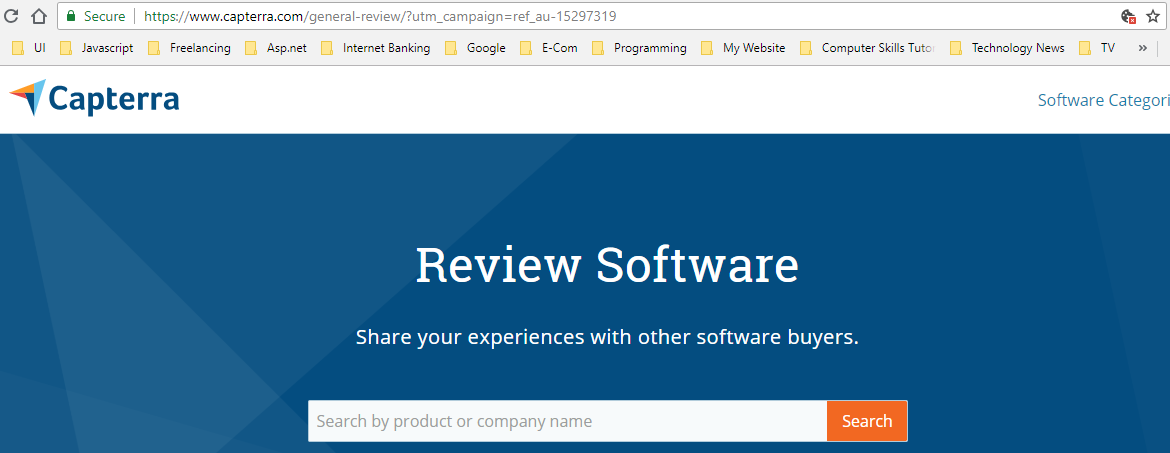This is a detailed screenshot of a web browser displaying a specific webpage. At the very top, there is a white address bar containing the website's URL. On the left side of the address bar, a small lock icon is shown, accompanied by the word "Secure," indicating that the connection is encrypted. Following a vertical gray line, the URL is displayed in black font: "https://www.captrera.com/general-review/?utm_campaign=ref_au15297319."

At the end of the address bar, there is a star icon which allows users to bookmark or favorite the website. Directly below the address bar, there is a gray toolbar displaying the user's bookmark folders. Starting from the left, the folders are organized as follows: "UI," "JavaScript," "Freelancing," "ASP.net," "Internet Banking," "Google," "EECOM," "Programming," "My Website," "Computer Skills Tutorial," "Technology News," and "TV."